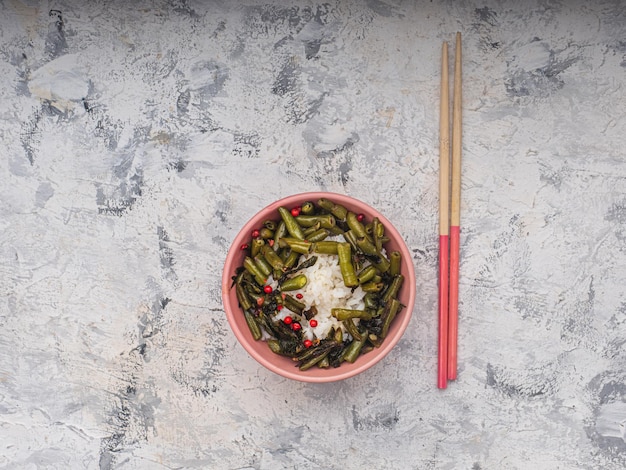The image features a vibrant and appetizing dish. At the center, a coral-colored bowl holds a serving of white rice topped with sautéed green beans, accented by small, red spherical objects that may be pink peppercorns or pomegranate seeds, adding both flavor and visual interest. On the right side of the bowl, a pair of wooden chopsticks with pink-tinted bottoms sit, their tips pointing upwards. The background is a swirling pattern of gray and white resembling a marble design, complementing the overall aesthetic. The combination of colors and textures in this scene creates a visually appealing culinary presentation.